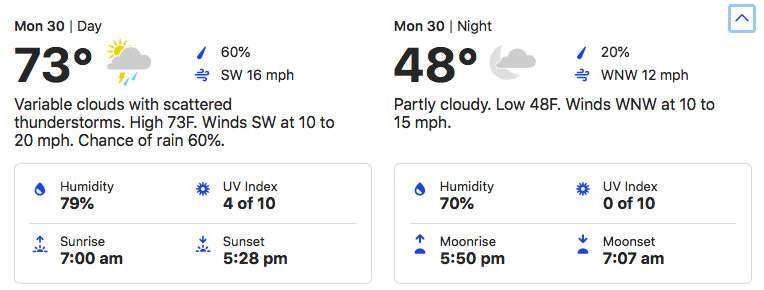Weather Forecast for Monday, October 30th

Day Summary:
- Date: MON30 
- Weather: Variable clouds with scattered thunderstorms
- Temperature: High of 73°F
- Icon Description: Sun partially obscured by a cloud, with blue and yellow raindrops beneath
- Chance of Rain: 60% (indicated by a blue raindrop)
- Wind: Southwest at 16 MPH
- Detailed Adaptation: Winds SW at 10 to 20 MPH
- Humidity: 79% (indicated by a half-blue, half-white drop within a gray-outlined rectangle)
- UV Index: 4 out of 10
- Sunrise: 7:00 AM (depicted with a sun and blue upward arrow)
- Sunset: 5:28 PM (illustrated with a sun and downward arrow)

Night Summary:
- Date: MON30 
- Weather: Partly cloudy
- Temperature: Low of 48°F
- Icon Description: Cloud and moon
- Chance of Rain: 20% (indicated by a drop)
- Wind: West-northwest at 12 MPH
- Detailed Adaptation: Winds WNW at 10 to 15 MPH
- Humidity: 70% (indicated by a half-white, half-blue drop within a gray-outlined rectangle)
- UV Index: 0 out of 10
- Moonrise: 5:50 PM (shown as a half-circle with an upward arrow)
- Moonset: 7:07 AM (depicted as a half-circle with a downward arrow)